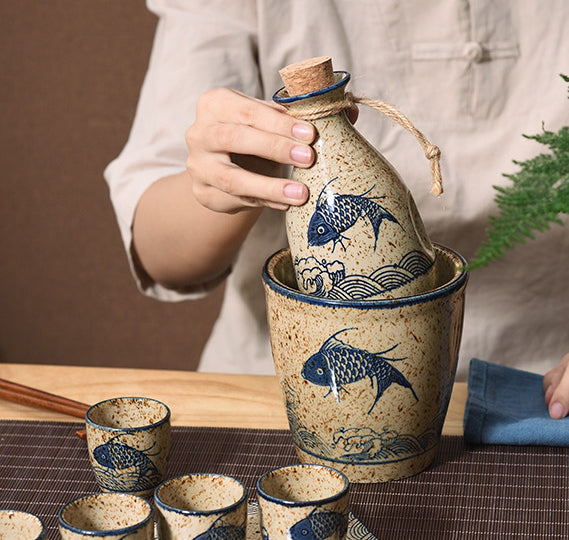In this detailed photograph, a person is holding a clay pot with a blue koi fish design, wearing a tan-colored apron and standing in front of a brown wall. The pot, adorned with a cork stopper and burlap twine, features a blue koi fish leaping over blue waves on a cream-colored base. The pot is being pulled out of a larger ceramic bowl with an identical design, possibly used to regulate temperature, suggesting this is a sake set. To the left of the bowl, a tray holds three small sake cups, and two more cups are positioned nearby, all matching the pot's design. A pair of chopsticks lies on the table's bamboo mat, which has a brown hue, adding a rustic touch. On the right, a denim-colored napkin and a small fern leaf add to the scene's aesthetic, enhancing the overall composition.